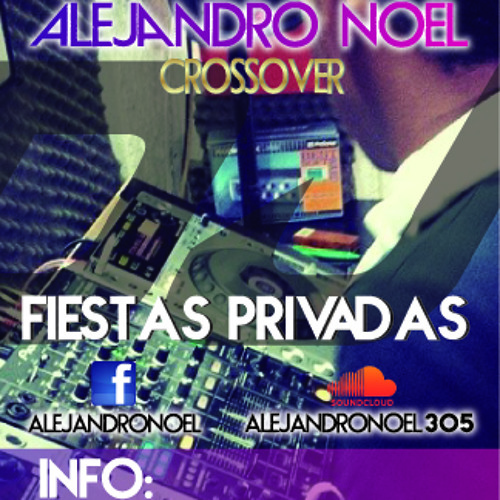The image is a colorful advertisement featuring an African American male DJ dressed in a black sports coat and white collared shirt, seated at a mixing board filled with various knobs and buttons. The scene appears to be a DJ booth, likely at a concert, with an array of DJ equipment visible, including a computer or screen displaying multiple colors like purple, white, black, and red. 

The text on the poster features a top section with "Alejandro Noel" written in a gradient that transitions from blue to purple, intended to give a neon-like effect. Below this, the word "CROSSOVER" is prominently displayed in gold, capital letters. Further down, in white text, you see "Fiestas Privadas." The bottom left corner includes a blue Facebook logo with a lowercase "f," followed by the Facebook handle "Alejandro Noel." Adjacent to this is a SoundCloud logo, featuring the handle "AlejandroNoel305." 

Additionally, at the very bottom of the advertisement is a transparent purple border, inside of which, in all cap white text, reads "INFO:" followed by an empty space. The background of the entire poster features the DJ at his turntables, actively performing, with elements like a red cloud-like base and a purple stripe pattern adding to the vibrant aesthetic.